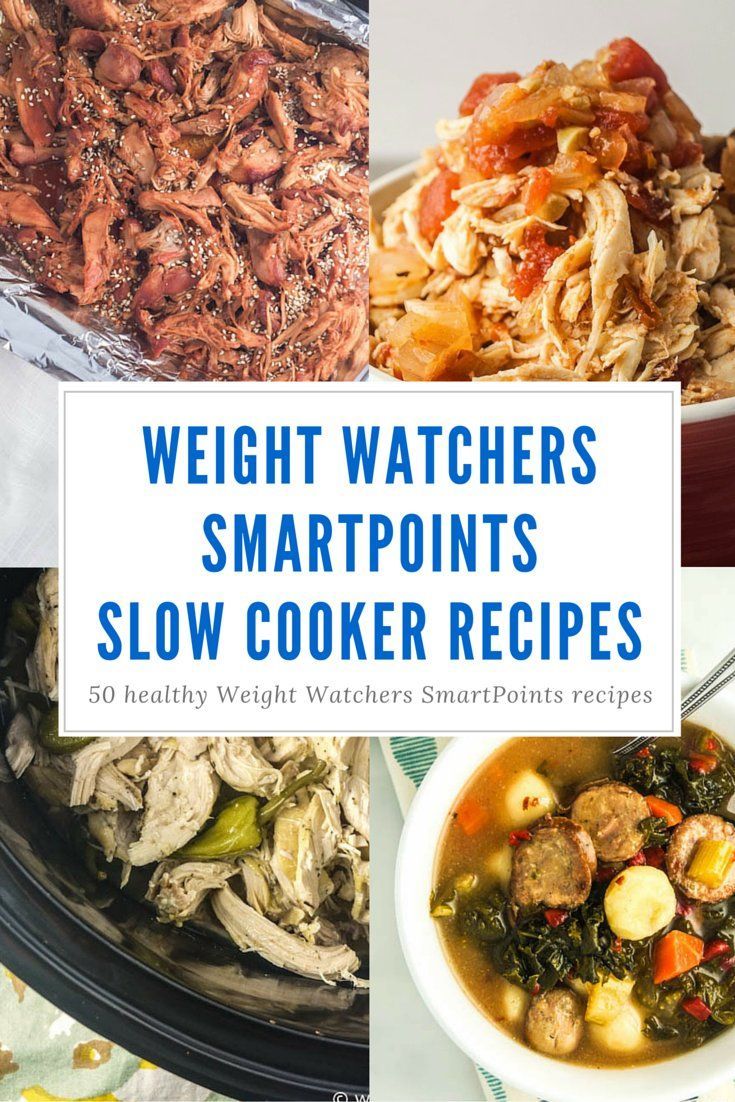This vertically oriented image depicts the cover of a recipe book titled "Weight Watchers SmartPoints Slow Cooker Recipes." The cover is divided into four quadrants, each showcasing a different dish photograph. Across the center of the cover, a large white rectangle with blue capitalized text reads "Weight Watchers SmartPoints Slow Cooker Recipes," and underneath in smaller dark text, it says "50 Healthy Weight Watchers SmartPoints Recipes." 

The upper left quadrant features an image of pulled pork, possibly in a pan or dish. The upper right quadrant displays roasted chicken with a colorful assortment of red and yellow vegetables. The lower left quadrant shows a black dish containing chicken pieces alongside a green pepper. Finally, the lower right quadrant portrays a hearty soup with sausage, potatoes, kale, and other vegetables like carrots.